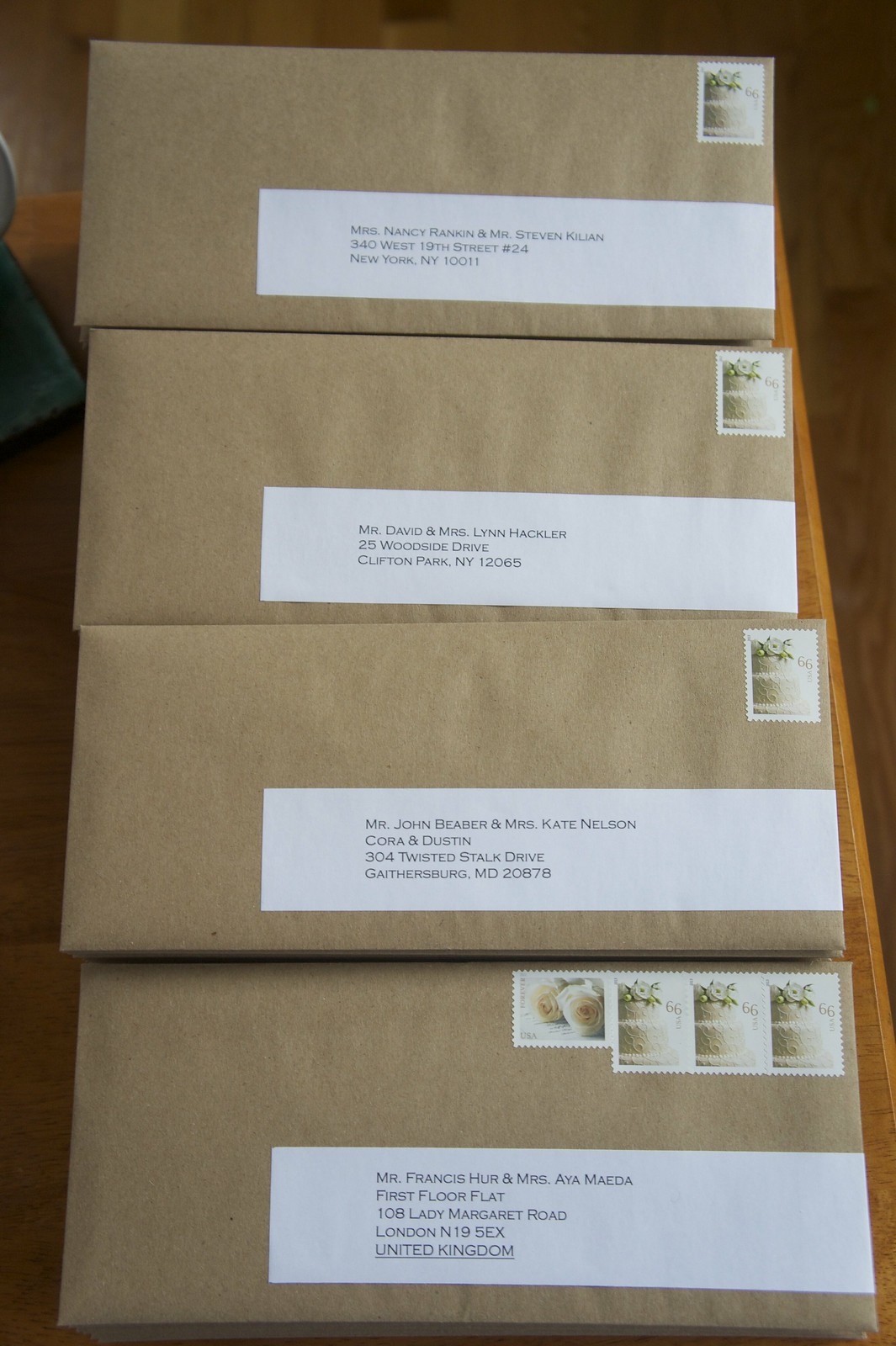The image depicts four neatly arranged brown craft paper envelopes set in a vertical column on a light brown wooden table. Each envelope is adorned with large white address labels, displaying the recipients' names and addresses. The top two envelopes are destined for New York: one addressed to Mr. David and Miss Lynn Heckler at 25 Woodside Drive, Clifton Park, NY 12065, and the other addressed to a couple in New York City. The third envelope is for Mr. John Barber and Ms. Kate Nelson at 304 Twisted Stack Drive, Gaithersburg, MD 20878, while the bottom envelope is headed to London, addressed to Mr. Francis Herb and Mrs. Jane Herb at 108 Lady Margaret Road, London N19 5EX, United Kingdom. The stamps on the envelopes include a wedding cake design with varying quantities: the top three envelopes each have a single stamp, while the bottom one features three wedding cake stamps and one depicting roses. The stamps are consistently placed on the top right corners of the envelopes, further adding to the meticulous, professional presentation of the parcels.